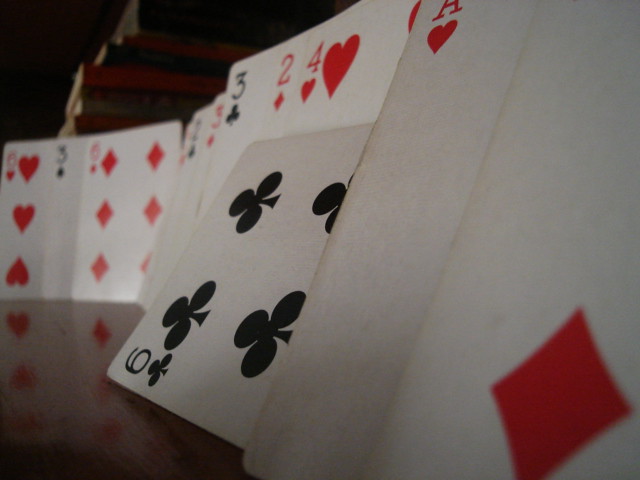The image captures a close-up view of a deck of playing cards, meticulously arranged upright on a highly polished wooden surface. The glossy finish of the wood creates a mirror-like reflection of the cards, adding depth to the composition. From left to right, the first card displayed is the six of hearts, followed by the three of spades. Next in line is the six of diamonds, with subsequent cards showcasing various numbers and suits, meticulously aligned in a cascading domino effect. In the forefront of the image, lying sideways, is the six of clubs, adding an intriguing element to the otherwise neatly lined collection. The careful arrangement and the reflective surface create a visually engaging scene, emphasizing the intricate details of the playing cards and the texture of the wooden surface.